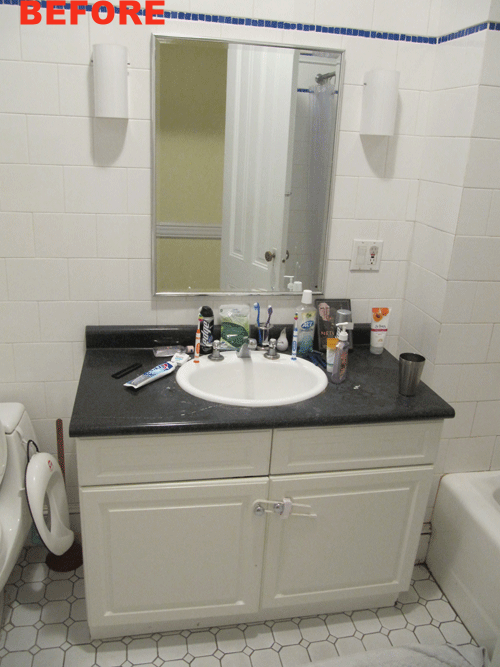This photograph captures a detailed view of a white-tiled bathroom. The wall tiles are predominantly white with a thin blue strip of tiles running horizontally near the ceiling. At the top of the image, the word "Before" is prominently displayed in red text.

At the center of the photograph, there is a mirror mounted above the sink, reflecting a white door and part of another wall. Flanking the mirror are two white sconces. Below the mirror, there is a white sink basin set into a dark gray countertop that appears slightly dirty, with visible white toothpaste stains giving it a dingy appearance.

On the countertop, to the left of the sink, sits a cup containing a purple and a blue toothbrush. Next to the cup is a light green and dark green bag, and beside it, a black, white, and silver canister. There is also an orange toothbrush lying next to the canister. To the right of the sink, there is a gray, blue, and white tube of toothpaste, accompanied by a small black object. Additionally, there is a clear bottle of mouthwash, a clear bottle of hand soap with a white top, a white and orange tube, and a silver cup.

Below the counter, white cabinets provide additional storage, and the floor consists of white tiles. On the left side of the image, there is a glimpse of a white toilet with a black plunger beside it. The right side of the image reveals a partial view of a white bathtub.